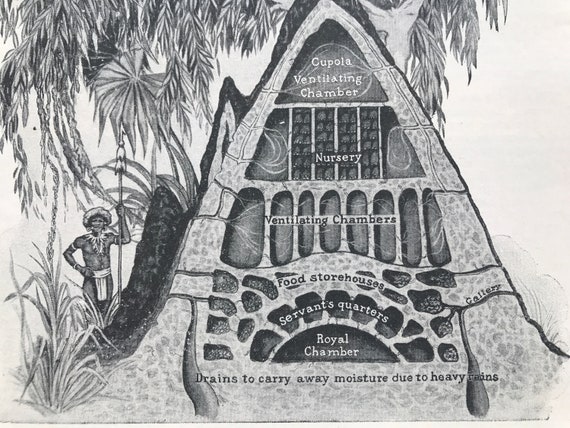This is a detailed black-and-white illustration depicting a cross-section of what appears to be an ant hill or termite mound. The structure is divided into various chambers, each labeled for its intended purpose. At the top, there is a "Coppola Ventilating Chamber," followed by a "Nursery." Further down, the mound contains additional "Ventilating Chambers," "Food Store Houses," "Servants' Quarters," a "Royal Chamber," and at the bottom, "Drains to Carry Away Moisture Due to Heavy Rains." To the left of the mound stands a figure, likely an Indigenous person, adorned in a loincloth and carrying a spear, reminiscent of Aztec or similar tribal attire. The scene also includes palm trees and other vegetation, adding to the contextual background of the illustration. This detailed diagram offers a fascinating glimpse into the hierarchical structure and functionality of the mound, with a clear emphasis on the various interconnected chambers and their specific roles.